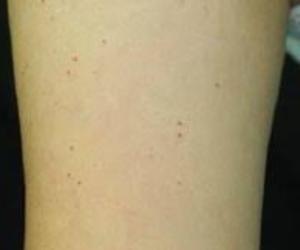The photograph is a close-up image of what appears to be a part of a human body, either an upper arm, forearm, or possibly a thigh. The skin is Caucasian, smooth, and relatively free of hair, suggesting it could be either the underside of a forearm or a shaven leg. The background of the image is dark, likely black, providing a stark contrast that emphasizes the details of the skin. The skin features several small, brown blemishes or spots, which may be moles, freckles, or signs of a mild skin condition such as psoriasis. The quality of the photo isn't very high, making some details less discernible, but the overall impression is of a normal, healthy limb with some minor skin markings.